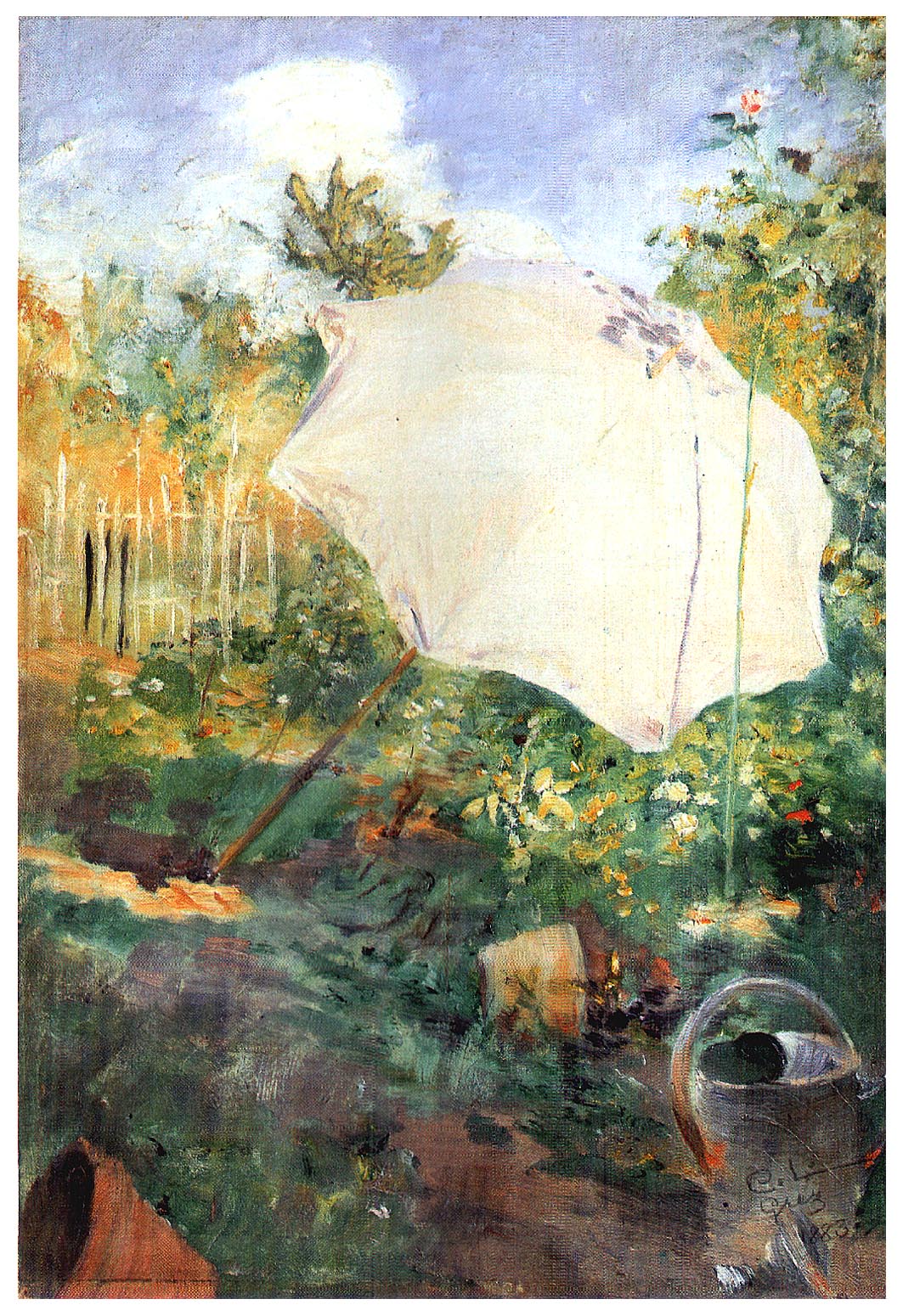The painting titled "Garden in Grez" by Carl Larson captures a serene yet subtly chaotic garden scene. Central to the composition is a white umbrella with floral designs, angled at 45 degrees, rooted firmly into the ground amongst patches of grass and flowers. The pastoral background showcases a crisp blue sky with scattered white clouds and a few trees. Midway through the scene, a rustic handmade fence composed of available sticks adds to the quaint atmosphere. In the foreground, there are a few scattered objects including a brown pot overturned on its side to the lower left, a silver bucket to the lower right, and a sprinkling can, suggesting a garden in the midst of work. The scene is painted in a Monet-esque style with soft, indistinct edges and a predominant color palette of greens and blues, which enhances its abstract quality. The oil painting technique emphasizes the texture and depth, making the garden appear both realistic and somewhat abstract.